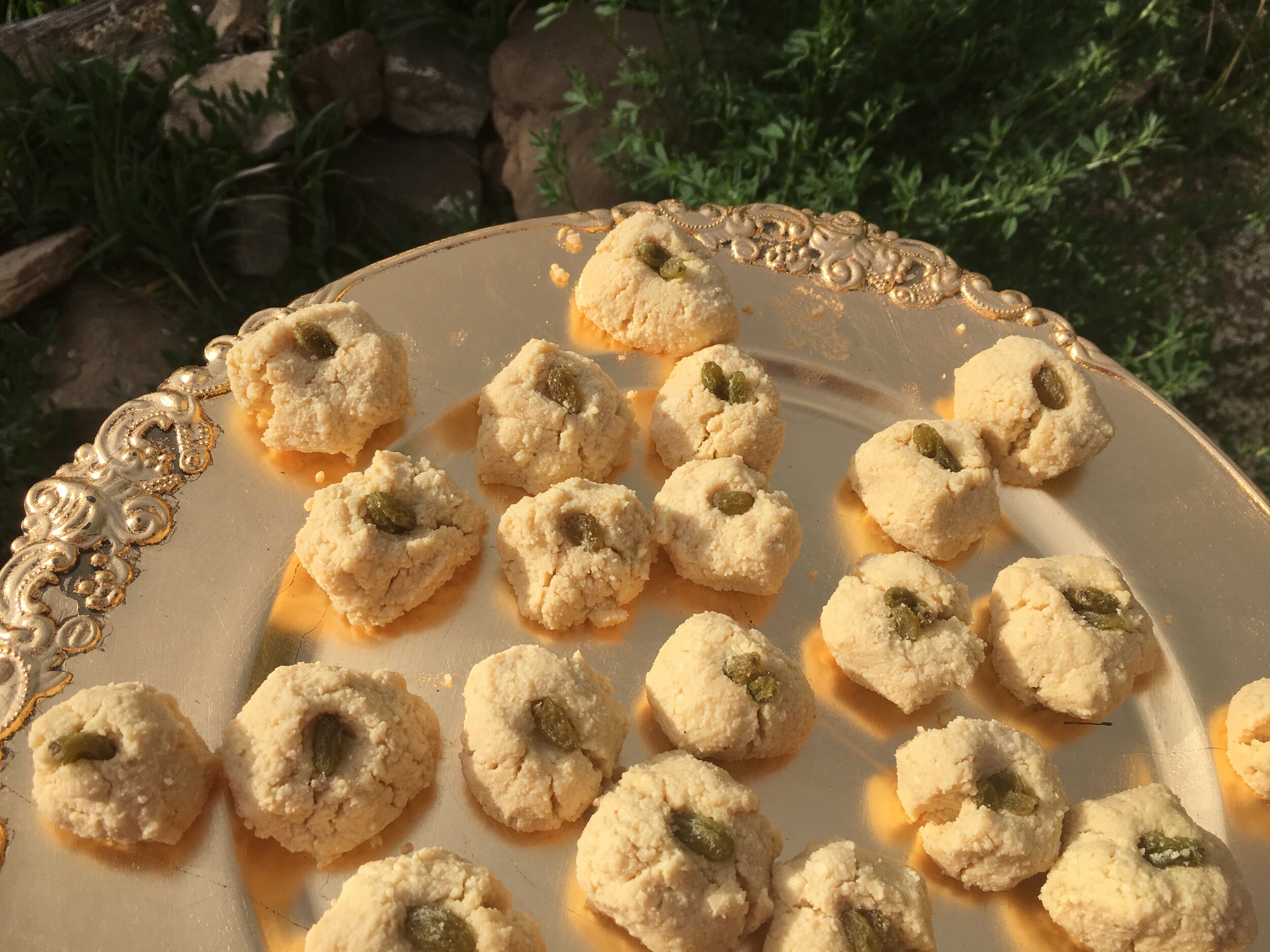A detailed photograph captures a bronze-colored plate with intricate engravings around its edges and left side, laden with approximately 15-20 circular brown cookies or biscuits. Each cookie features a distinctive crinkled top, with a single light green nut, likely a pistachio, pressed into its center. The cookies are arranged randomly across the plate. Surrounding the plate, there is some green leafy material, suggesting the presence of ferns or ivy, and the rocks in the background hint at an outdoor setting. The photo is taken from a slightly angled top-down perspective, focusing on the finely detailed platter and cookies. There are no signs of human involvement, and the scene is devoid of any text or words. The whole arrangement exudes an air of elegance and simplicity.